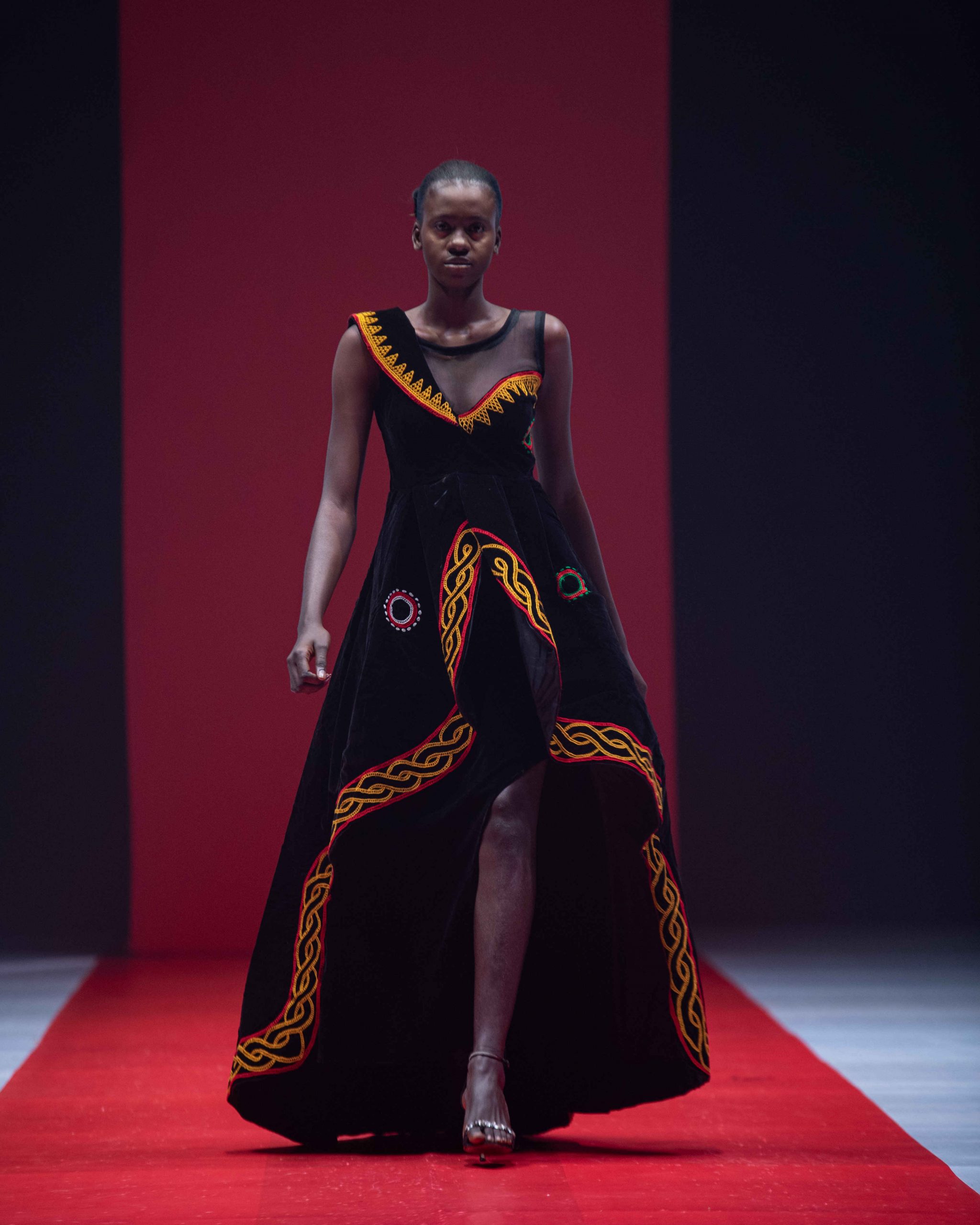A tall, slender African woman is centrally positioned in this photograph as she elegantly walks down a red carpet runway during a fashion show. Her skin, rich and dark like chocolate, contrasts beautifully with her attire and the setting. She wears a striking black dress adorned with gold trim along the neckline and hem, and the dress reveals her left leg with a low-cut design. Her short, possibly closely shaved black hair, adds to her poised and graceful presence. Her arms are at her sides, but her right arm swings slightly forward in sync with her left leg, capturing the fluidity of her stride. On her feet, she's wearing delicate sandal-like shoes featuring thin horizontal loops near her toes and ankles, embellished with small gems that glisten subtly against the spotlight. The runway floor is a gray hue, while the background is dominated by a red curtain that mirrors the width of the carpet, completing the vivid and professional atmosphere of this fashion show.